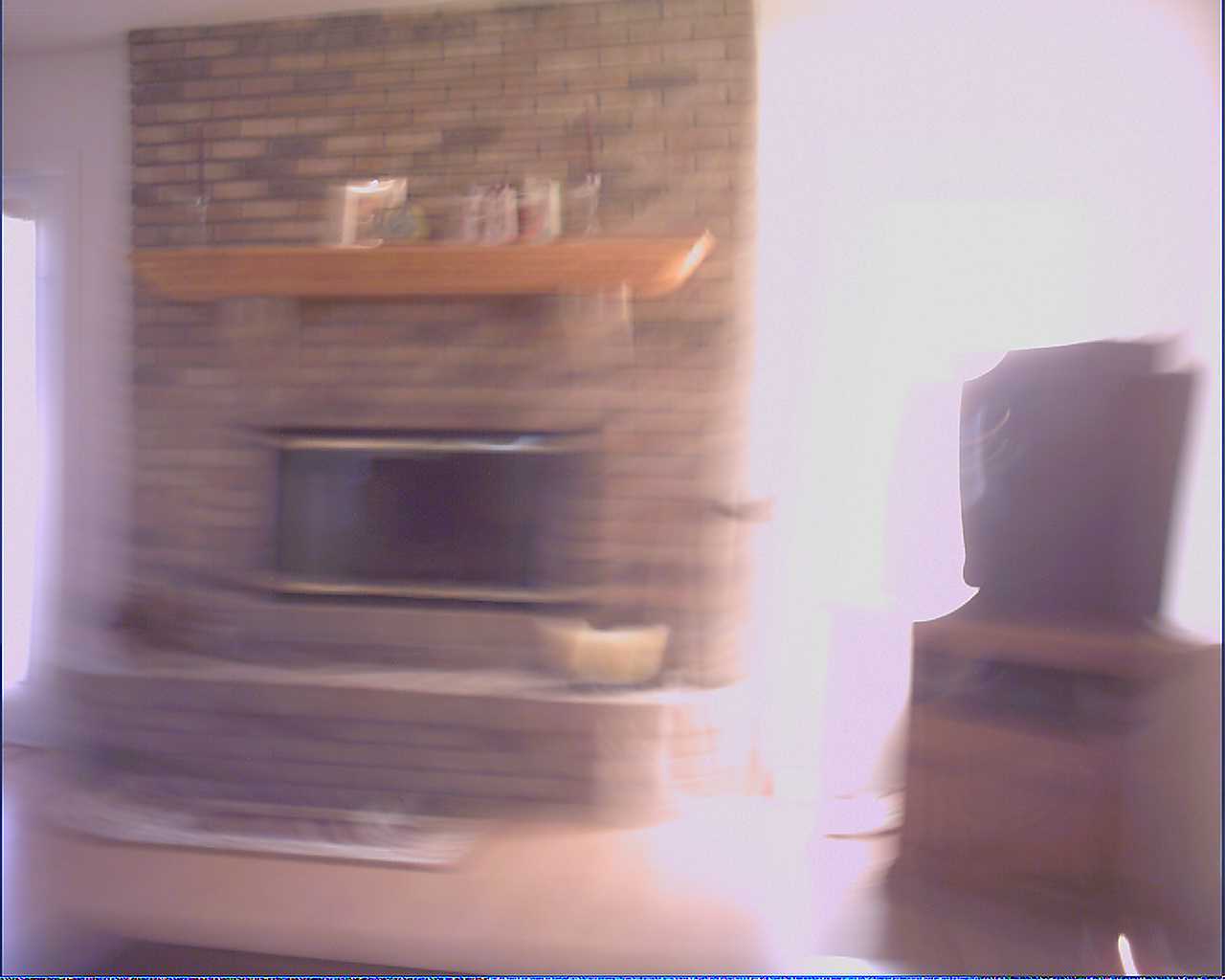This photograph, likely taken accidentally, is an extremely blurry and low-quality image, reminiscent of those that end up on your phone's camera roll by mistake. The scene appears to be a living room with a prominent brick fireplace as the central focus. The fireplace, constructed of yellow, brown, and cream-colored bricks, features a wide rectangular opening with reflective goldish bands suggesting a metallic trim. Extending from the fireplace is a hearth, about a foot and a half high and extending one to two feet outward, adorned with a basket and other indistinguishable items, possibly tools for stoking the fire. In front of the hearth lies what might be a dog bed or a rug. 

Above the fireplace, a wooden mantle is mounted, supported by some of the brickwork and holding various objects, including picture frames. To the right side of the image, albeit very blurry due to a bright light, there seems to be a wooden TV stand with a TV or black object on top. The light streaming in from this side further blows out details, making the right third of the photo even harder to decipher. Overall, the image is marked by poor contrast, excessive brightness in certain areas, and an overall grainy, motion-blurred quality that obscures finer details.